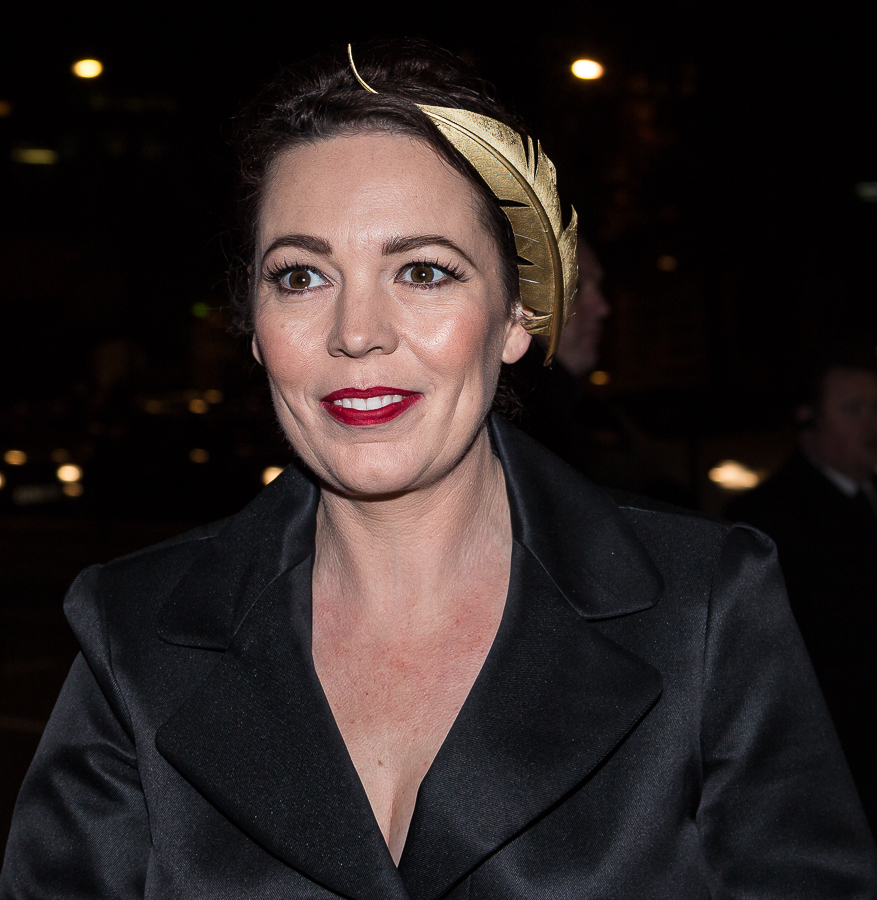This image captures a middle-aged woman, likely in her 40s, at a high-profile event, suggesting a paparazzi or press photograph taken at a party. She has an unmistakable look of familiarity, dark brown hair gathered and adorned with a large, gold feather hair accessory on her left side which curves around her hair and drapes behind her ear. Her deep brown eyes and red lipstick highlight her prominent cheekbones, giving her a slightly surprised yet smiling expression with rosy cheeks and forehead. She is dressed in a shiny black blazer with exaggerated lapels that form a V-neck, although nothing underneath is visible. The backdrop is predominantly dark with scattered yellow lights suggesting an event setting, and you can make out some people mingling in the background, adding to the ambiance of the image.